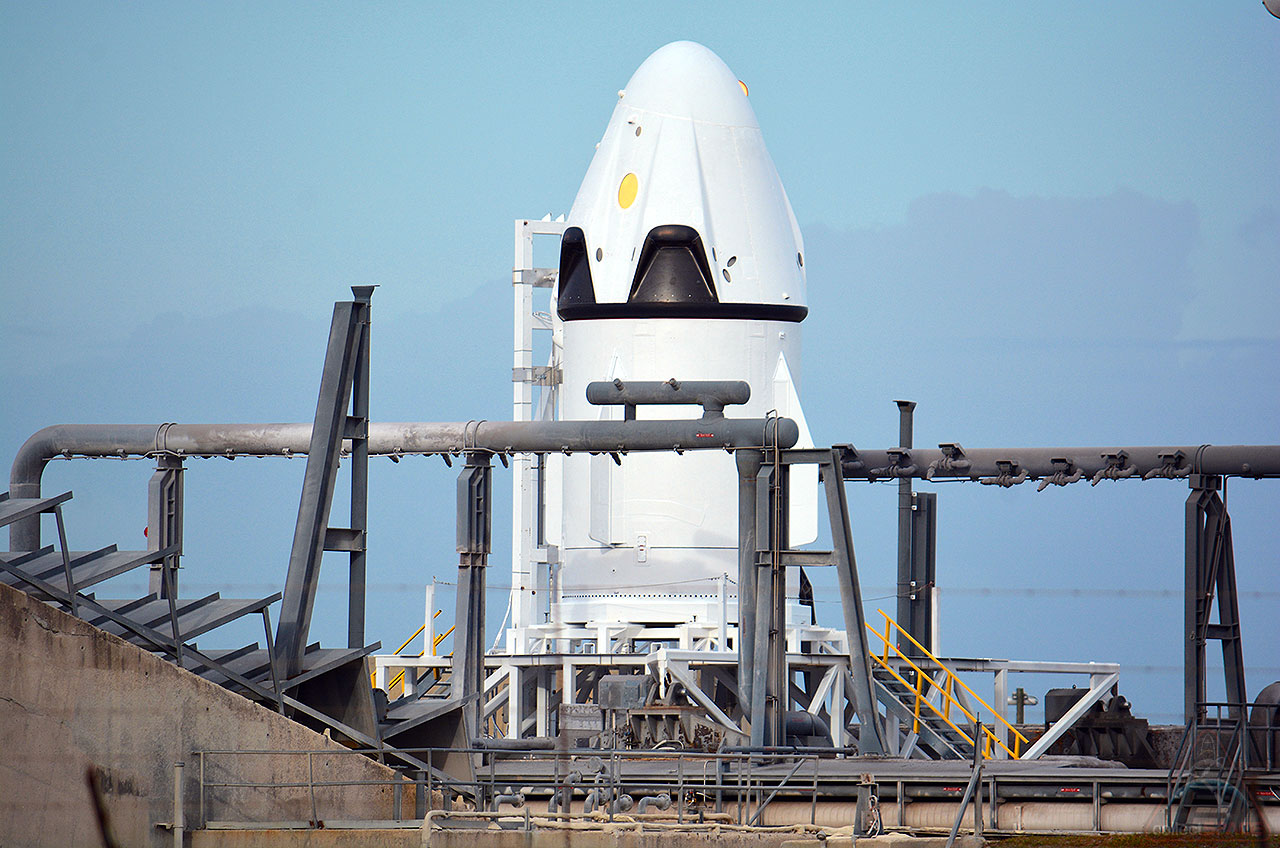The image features a white rocket prominently positioned in the center, set against a completely clear blue sky. The rocket's cylindrical body transitions into a cone-shaped upper part, characterized by a black band around it and several black windows or doors near the top. There is also a distinct yellow circle on the rocket's exterior. Surrounding the rocket is a complex launch platform structure, predominantly metallic and gray. In front of the rocket, a horizontal gray pole and some supporting stands are visible. To the left of the platform, a flight of metal stairs with yellow handrails leads up to a base. The foreground features more metallic elements and some brown areas, likely part of the launch apparatus. No people or text are visible in the image. In the far background, there are indistinct and barely visible buildings.